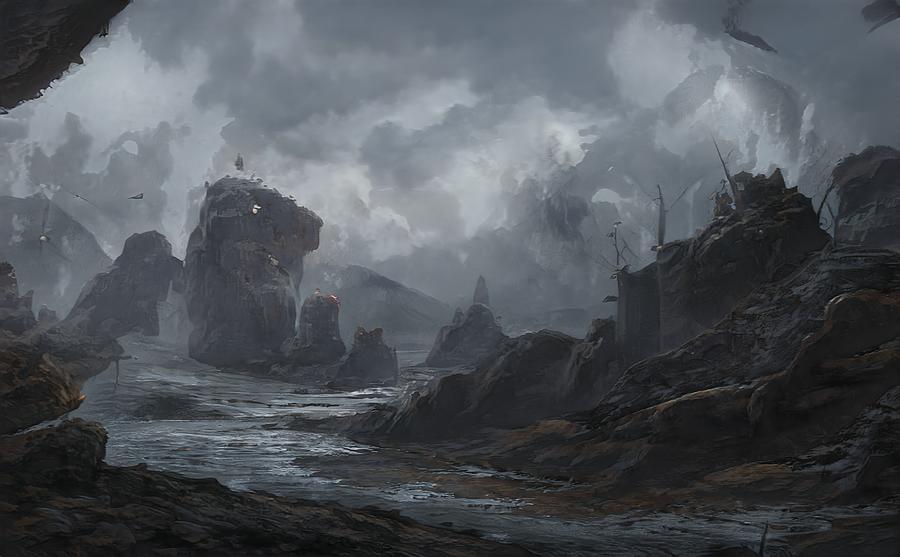The image depicts a moody, dark scene characteristic of a graphic novel or a prototype for a film. It showcases a sparse, rocky coastline with jagged rocks jutting out of the water, suggesting a very low tide. The atmosphere is brooding with a heavy, cloudy sky that has a digital appearance, encompassing shades of grey, light, and dark. The water in the scene appears to have receded, revealing brown vegetation and barren flat areas near the bottom left corner. Mountains loom in the background, adding to the secluded and desolate feel. On the right side, sheer cliff walls are visible, topped with some kind of equipment. Pointy objects protrude from the rocks, though it's unclear whether they are natural formations or man-made structures. In the top right corner, a couple of birds can be seen, adding a sparse touch of life. The overall hyper-realistic image creates a somber, almost otherworldly landscape.